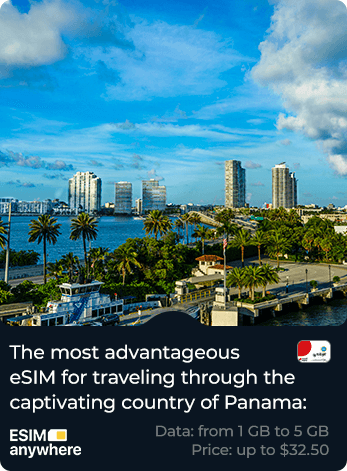**Caption:**

This vibrant advertisement, possibly designed for a website, features a large rectangular image with rounded corners that beautifully showcases the allure of Panama. The bottom third of the image is dominated by a black bar with left-justified white text, highlighting the product's benefits: "The most advantageous eSIM for traveling through the captivating country of Panama." To the right of this text, a small white rectangle symbol with a distinctive red semicircle in the top-left corner provides a visual cue, although its finer details are too small to discern.

In the bottom-left corner of the black bar, the words "eSIM Anywhere" accompany a drawing of a SIM card, emphasizing the service's accessibility. The bottom-right corner lists the data options in pale grey text: "Data: from 1 GB to 5 GB, Price: up to $32.50."

Above this informative section, the advertisement boasts a very colorful and vibrant photograph presumed to be of a Panamanian landscape. The image captures the beauty of the sea, surrounded by numerous palm trees, distant buildings, and impressive skyscrapers. The bright blue sky, interspersed with wispy white and occasional grey clouds, complements the picturesque scenery, making it an inviting glimpse of Panama's captivating environment.